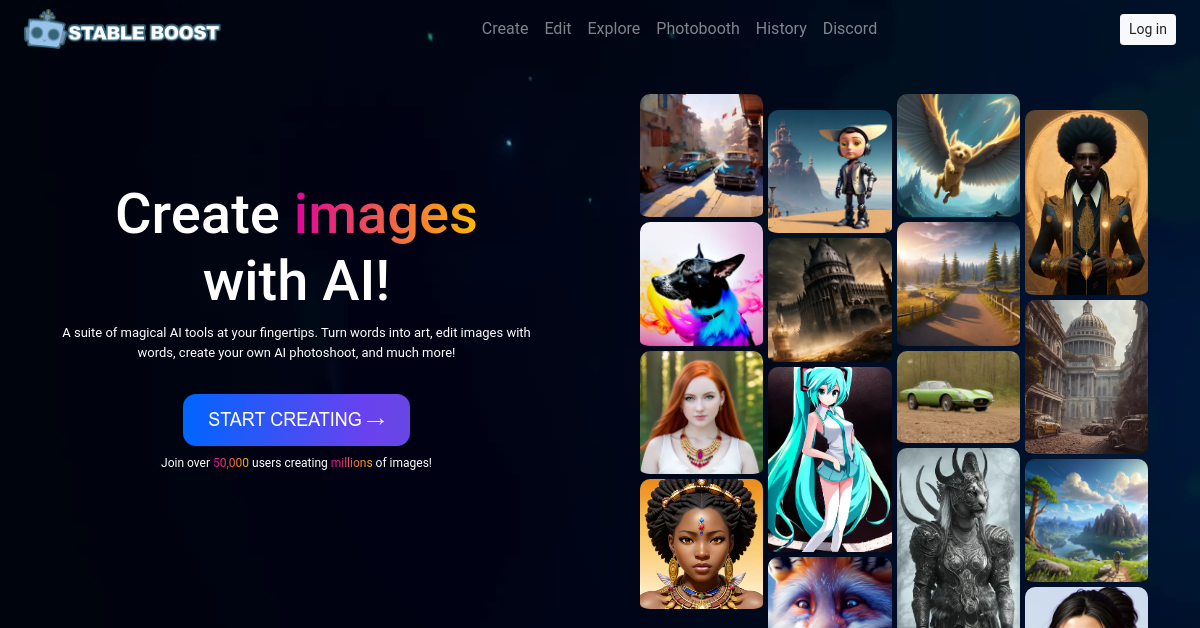The image displays a webpage featuring a colorful collage of images depicting various people and places. In the upper left corner, the text "Stable Boost" is prominently displayed. The background of the webpage is black, providing a stark contrast to the vibrant visuals.

At the top of the page, there are several navigation sections labeled: Create, Edit, Explore, Photo Booth, History, Discord, and Login. A white login button is also visible. On the left side of the page, there is descriptive text inviting users to "Create images with AI." The word "images" is highlighted in a gradient of pink and orange, and the accompanying text reads, "A suite of magical AI tools at your fingertips. Turn words into art, edit images with words, create your own AI Photoshop, and much more." Below this description is a prominent blue button labeled "Start Creating," with a call to action inviting users to join over 50,000 others who are collectively generating millions of images.

To the right, there are various example images showcasing the capabilities of the AI, including images of cars, mystical creatures, dogs, and people dressed as fairies, among other imaginative designs. Among these, there is a noticeable image of a woman with striking red hair and another of a woman who resembles an African queen, both in elaborate costumes and settings.

Overall, the website "Stable Boost" offers a platform for creating AI-generated images, and the layout and examples suggest a user-friendly, visually driven experience ripe with creative possibilities.